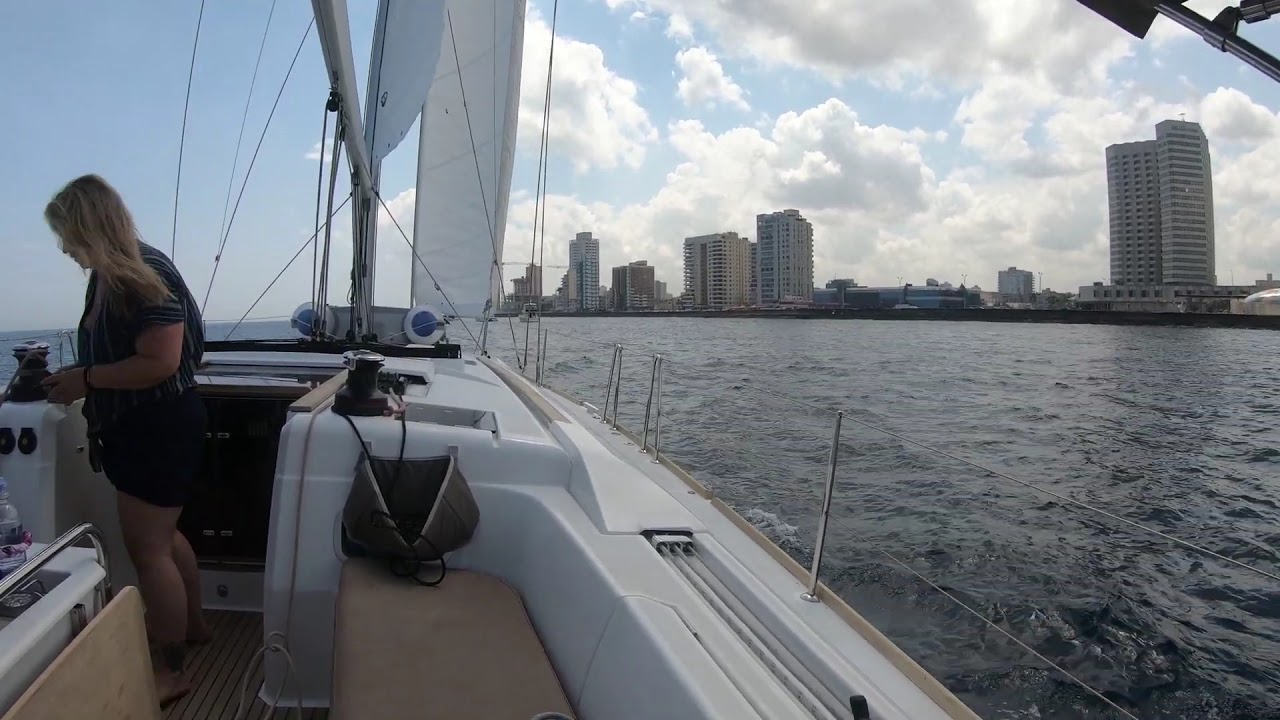A vibrant image captures a young woman with long blonde hair, wearing a black short-sleeve shirt and black shorts, standing on a tan and white sailboat. She appears to be focused, possibly handling a sailing wire or some other boat-related task. Detail of the boat includes a white sail prominently hoisted, coupled with visible lines and cushions. The scene is set against a backdrop of choppy waters, suggesting dynamic sailing conditions. The boat is sailing in a large harbor adjacent to a bustling cityscape, where numerous tall buildings, including several skyscrapers with many windows, stretch along the riverbank. The sky above features a mix of clear blue to the left and large, fluffy white clouds to the right, indicating a bright and lively midday atmosphere.